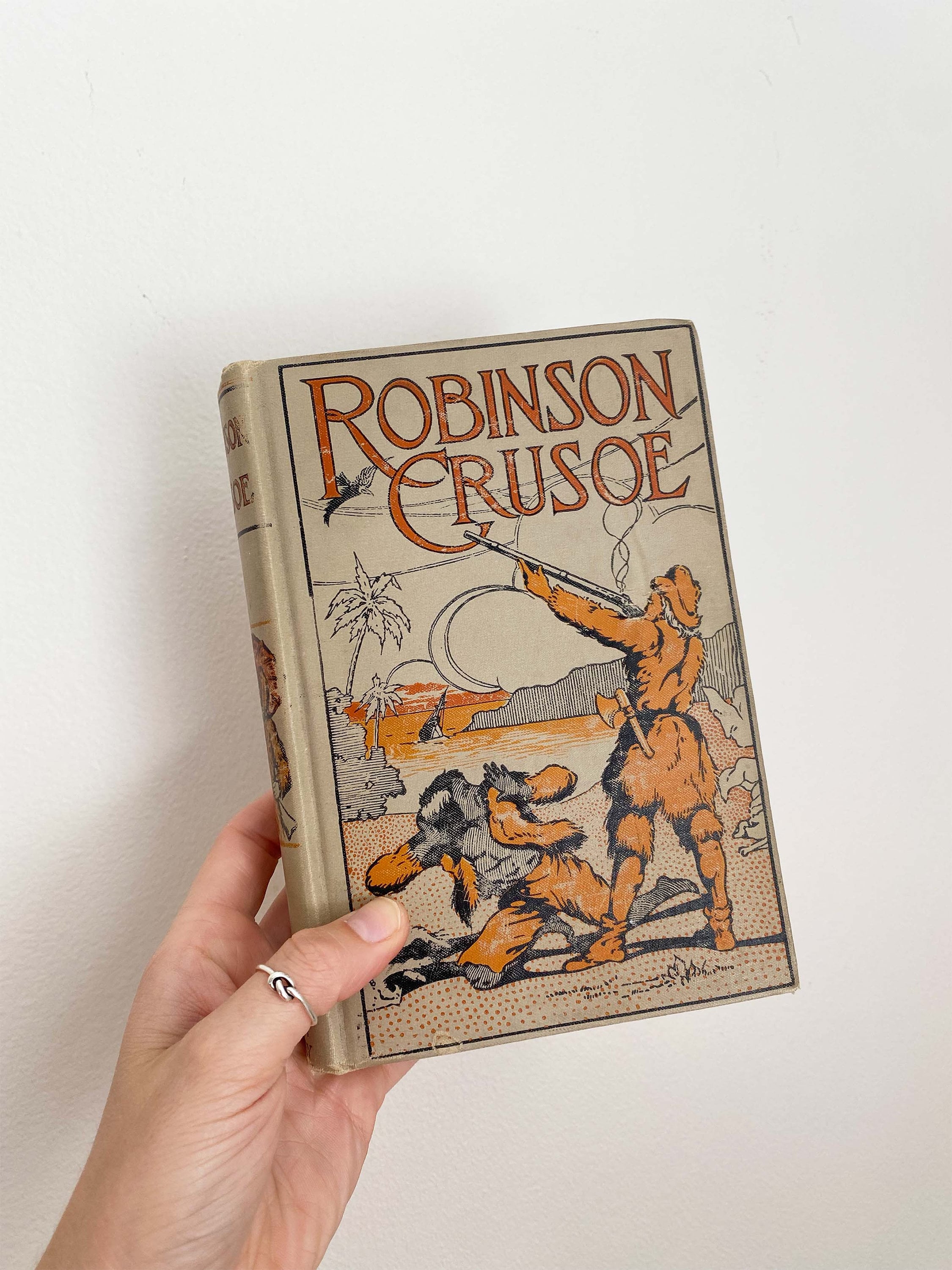In this detailed photograph, a woman's fair-skinned hand, adorned with a distinctive silver ring that loops into a knot, emerges prominently from the bottom left, holding up an older hardcover copy of "Robinson Crusoe" against a plain white wall. The hand is highly detailed, showcasing the lines of the palm and the creases where her fingers fold over the cover. The book itself is a grayish-beige color, slightly distressed, yet well-preserved. At the top, the title "Robinson Crusoe" is prominently displayed in bold, all-caps orange lettering with a black outline. The cover illustration is rendered in navy and orange, depicting a vivid scene: a man in a fur hat, fur jacket, and fur pants points a musket towards a bird in the sky, standing on a beach-like setting with an orange sea, palm trees, and a distant boat. In front of him, a darker-complexioned man wearing orange pants and an orange fur open jacket cowers on one knee. The book's spine, just barely visible, appears to match the cover's orange and navy blue color scheme.